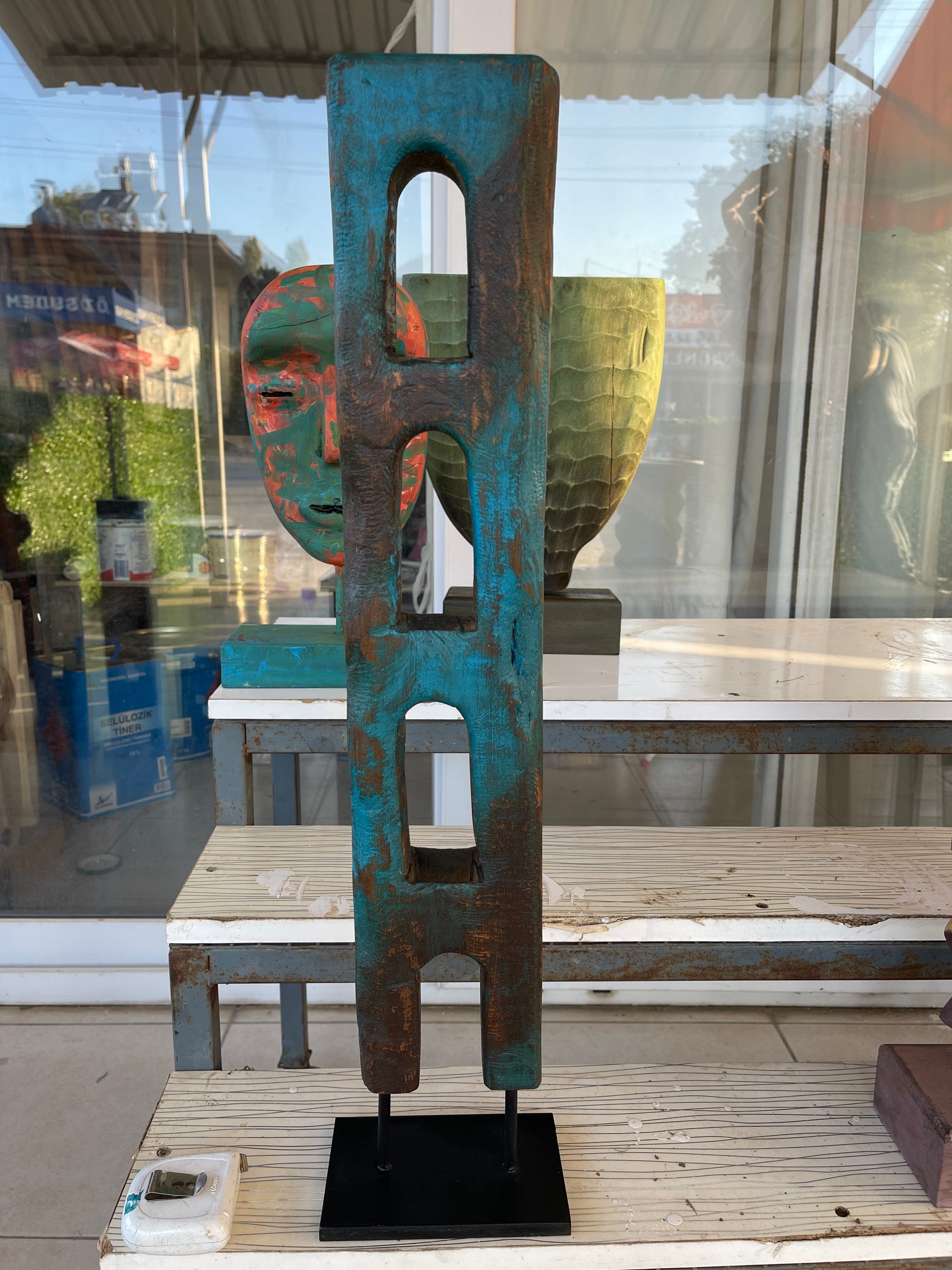This photograph captures an intricate and vibrant piece of art as its focal point. Central to the image, at the bottom, is a black rectangular base. Two slender black poles extend vertically from the center edges of this base, supporting a slightly elevated rectangle with a hollowed-out bottom center. This structure transitions into metal accents and an upward-reaching arched doorway. The metal is richly colored, featuring a gradient of bright blue merging into gray, with hints of orange, reminiscent of paint gracefully peeling away without visible chips.

This captivating art object is displayed on a white painted wooden shelf, itself part of a gray metal frame. The frame supports a series of shelves positioned behind the artwork, each progressively higher. Occupying the top shelf is an oblong mask, presented in vibrant shades of green and yellow. Adjacent to the mask, on the topmost shelf, is a large green vase, which gradates from a light green at the top to a grayish hue at the base.

The background is a striking floor-to-ceiling window, allowing reflections to softly dance across the glass, adding a subtle yet dynamic depth to the composition.